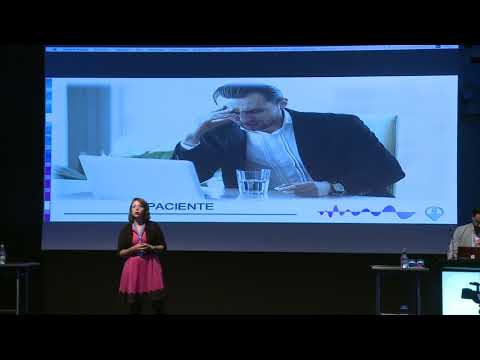The image captures a moment of a woman giving a presentation on stage in what appears to be a large auditorium. Positioned in the lower left corner of the image, the woman stands confidently, wearing a pink dress paired with a black sweater, a blue lanyard, and pink or red lipstick. She has dark brown hair and is speaking to the audience. Beside her, on the right, is a partial view of a desk or counter with another man sitting behind it, focused on his Apple laptop. This man, identified as possibly African-American, is wearing a gray shirt.

Dominating the background is a large projection screen displaying an image of a man sitting at a table, appearing stressed with his right hand pressed against his temple. The man is dressed in a black sports coat and a business shirt and has a glass of water and a laptop in front of him. The image on the screen suggests a theme of distress or concentration, which is likely tied to the presentation's topic. The scene captures a dynamic moment of interaction and communication, highlighted by the vivid colors and distinct details of the environment.